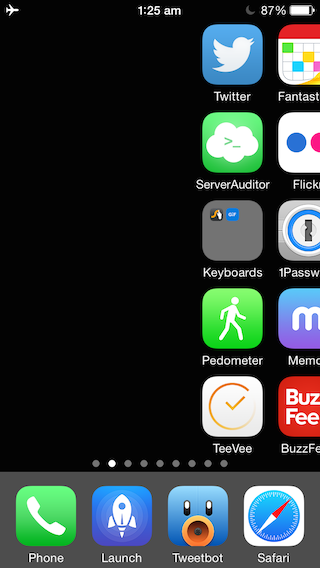This image is a detailed screenshot of a smartphone's home screen, specifically focusing on the app arrangement and status indicators. At the bottom dock of the screen, several apps are prominently displayed. From left to right, there's a Phone app, an app labeled "Launch" likely used for accessing more apps or websites, Tweetbot for managing Twitter posts, and the Safari browser.

The leftmost part of the screen is completely black, while the right side showcases various app icons arranged in a grid. Starting from the top left, the Twitter app is visible, followed by a gaming app to its immediate right. Below Twitter is the Server Auditor app, and to its right is the Flickr app. Underneath Server Auditor is a keyboard app, and next to this is the 1Password app, presumably a password manager. Below the keyboard app is a Pedometer app for tracking steps, with a Memos app to its right for jotting down notes and reminders.

Further down, a TV viewing app lies below the Pedometer app, and to its right is the BuzzFeed app, likely used for browsing social media content.

The status indicators at the top-left of the screen show that the phone is in Airplane Mode, as indicated by the airplane icon. The time reads 1:25 a.m., and the battery level is at 87% charge.

Overall, this screenshot provides a comprehensive view of the various apps the phone's owner uses for both work and leisure activities, along with essential status information.